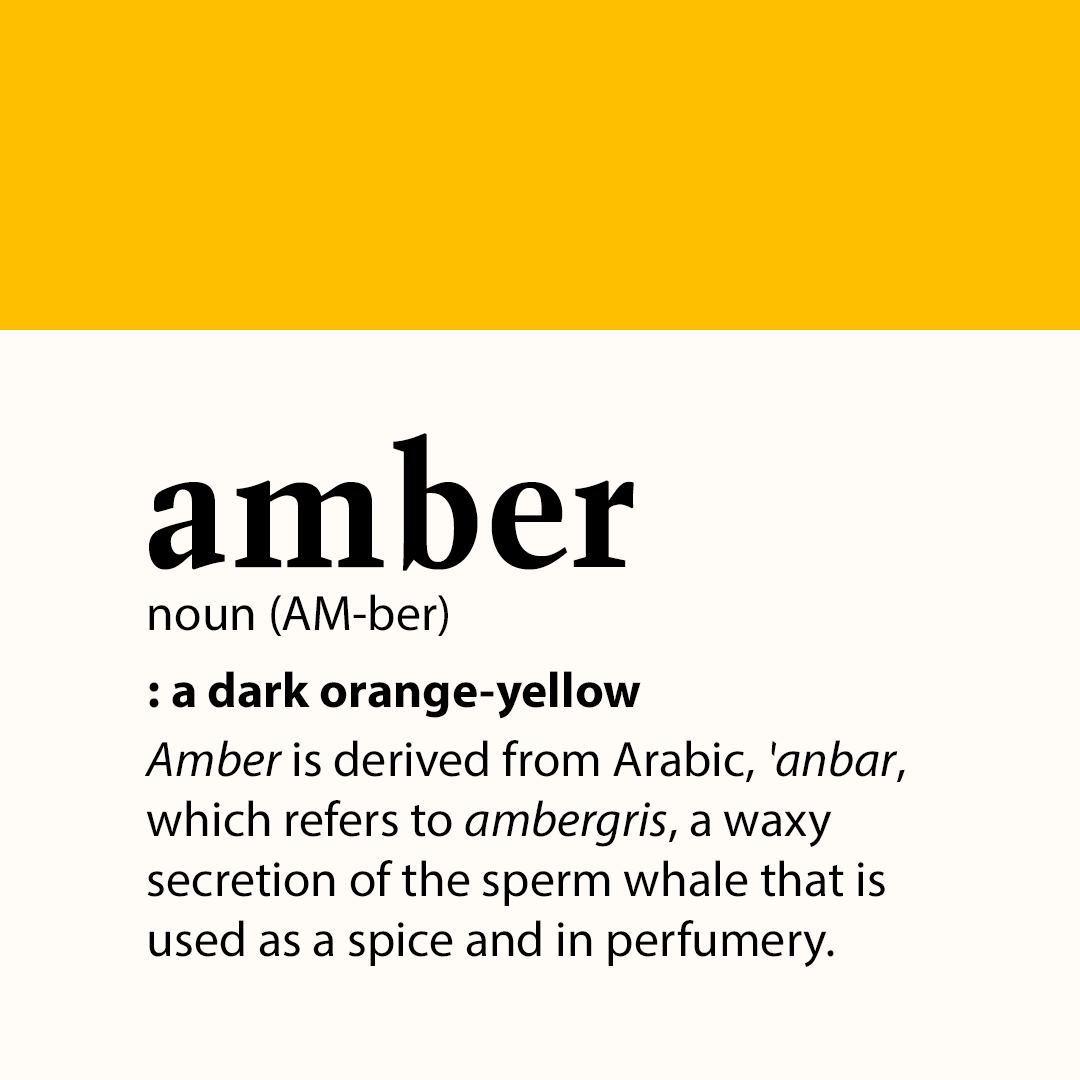The image is a detailed illustration set against a white background, featuring a color story. At the top of the square layout, there is a yellowish-orange stripe, sometimes described as mango yellow, or a yellow-green-orange color. Below this stripe is black text, prominently displaying the word "amber" in large lowercase letters. Beneath "amber," the word "noun" is listed, followed by the pronunciation "am-bur" in parentheses, with "am" in capital letters. The definition provided reads: "a dark orange-yellow." The text further explains that "amber" is derived from the Arabic word "anbar," referring to ambergris, a waxy secretion of the sperm whale used in spice and perfumery. The lower part of the square features a light beige background, enhancing the contrast with the text above.